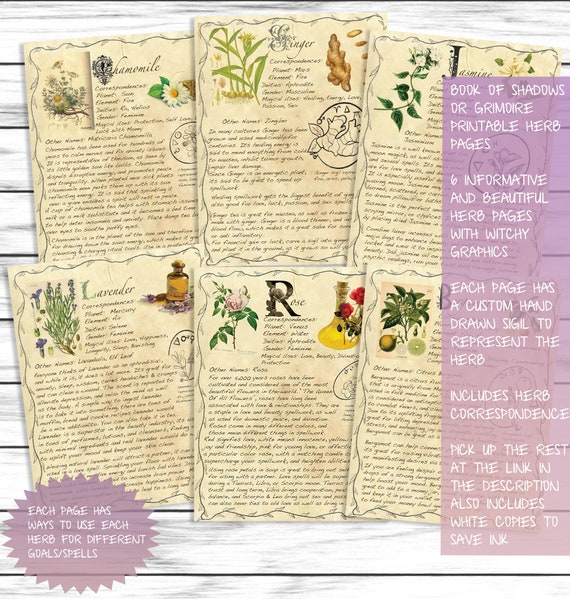This collage-style image features six digitally designed, aged parchment pages laid out in two rows of three against a textured gray and white wooden backdrop. Each page is meticulously crafted to resemble an old, yellowed document, complete with decorative, witchy graphics and a hand-drawn sigil representing the herb. The top left page is dedicated to Chamomile, followed by Ginger, Jasmine, Lavender, Rose, and an herb starting with the letter 'B.' 

Each herb page includes a vivid illustration of the plant in the upper left corner, followed by its name in elegant script. Below, there are extensive paragraphs detailing the herb's uses, correspondences, and applications in various goals or spells. On the right-hand side of the image, sections with a light purple background display titles in white text, promoting these as "Book of Shadows" or "Grimoire Printable Herb Pages". Additionally, a pink circular graphic with jagged edges emphasizes that each page is both "Informative and Beautiful," featuring detailed descriptions and custom sigils, specifically designed to save ink. The image invites viewers to explore more and complete their collection via a link provided.